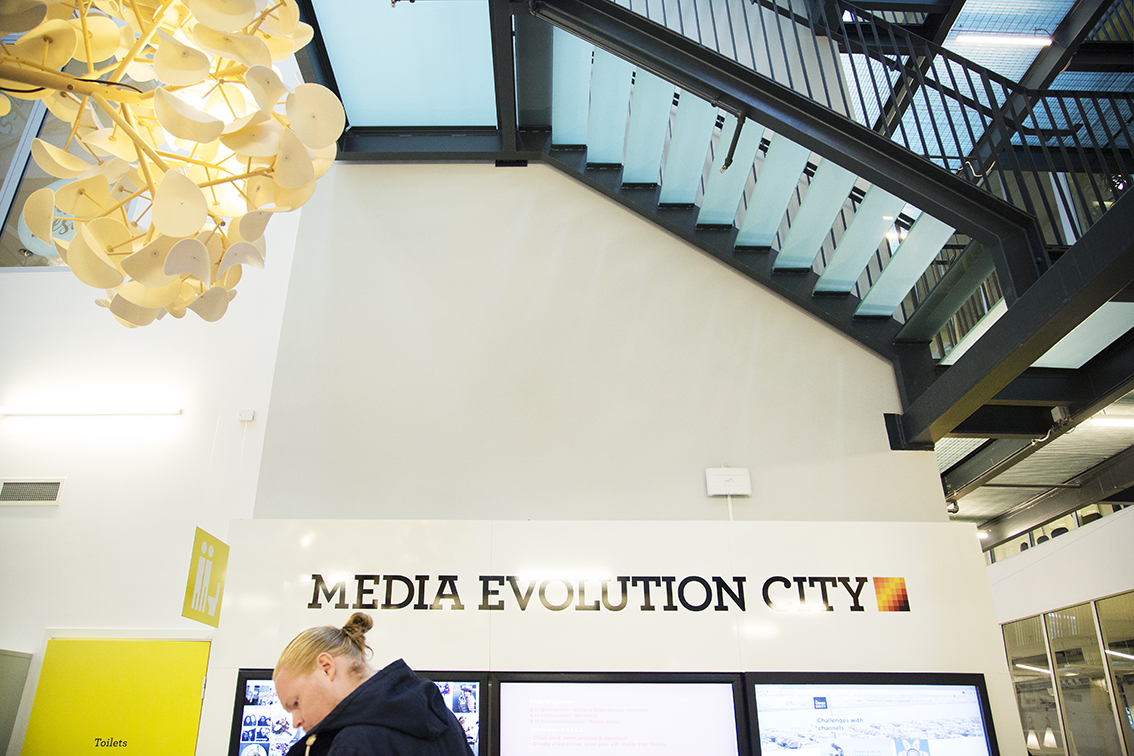The image depicts an indoor setting, likely within a government building or a college campus. Central to the composition is a sign that reads "Media Evolution City" in bold, black text accompanied by a logo featuring pixelated blocks in various colors. To the left, a woman with reddish blonde hair pulled into a messy bun is casually walking; she wears a black hoodie and appears to be gazing downward. Behind her, in the upper left corner, hangs a light fixture designed to resemble a plant, with circular, yellowish-white leaves. 

The upper right part of the image showcases an impressive glass staircase with light blue, slightly transparent steps, supported by sleek, black metal railings—a striking example of modern design. Dominating the right-hand side of the image is a bright yellow door labeled "Toilets," and a corresponding overhead sign indicating restroom facilities with icons of a man, a woman, and a toilet. The surroundings feature a blend of white, black, and various shades of blue, further enhanced by the light reflecting off the shiny surfaces and lending a contemporary yet casual atmosphere to the scene.